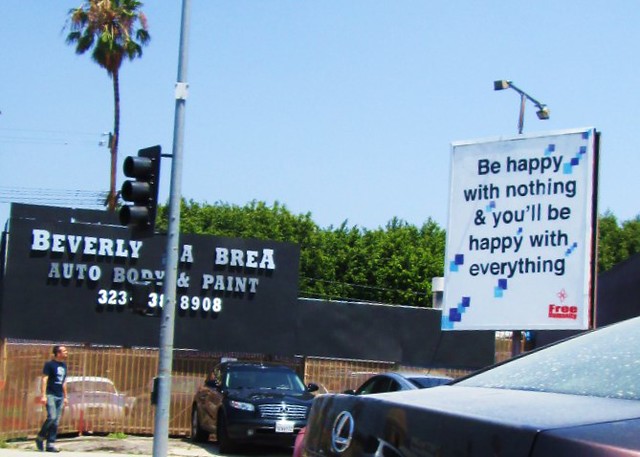This outdoor photograph captures a scene dominated by a well-composed juxtaposition of elements. 

Near the right side of the image, a prominent white sign with dark lettering reads: "Be happy with nothing and you'll be happy with everything." The sign is tastefully adorned with light and dark blue squared designs behind the text, providing a visually pleasing contrast. At the bottom right corner of this sign, red print declares "free."

To the left of the sign, a dark-colored building stands, featuring a brown fencing structure at its base, presumably encircling a parking area occupied by several cars. At the top of the building, in lighter letters, the words "Beverly & Brea Auto Body and Paint" are visible. Some parts of this sign on the building are obscured by a metal traffic signal pole equipped with black housing and three circular lights.

A man with blue jeans and a dark shirt is present in the foreground, adding a human element to the scene. Among the parked cars outside the building, various trees contribute to a natural backdrop, including lush, bushy trees and a notably tall palm or tropical tree. The sky overhead is a medium blue, suggesting a clear and pleasant day.